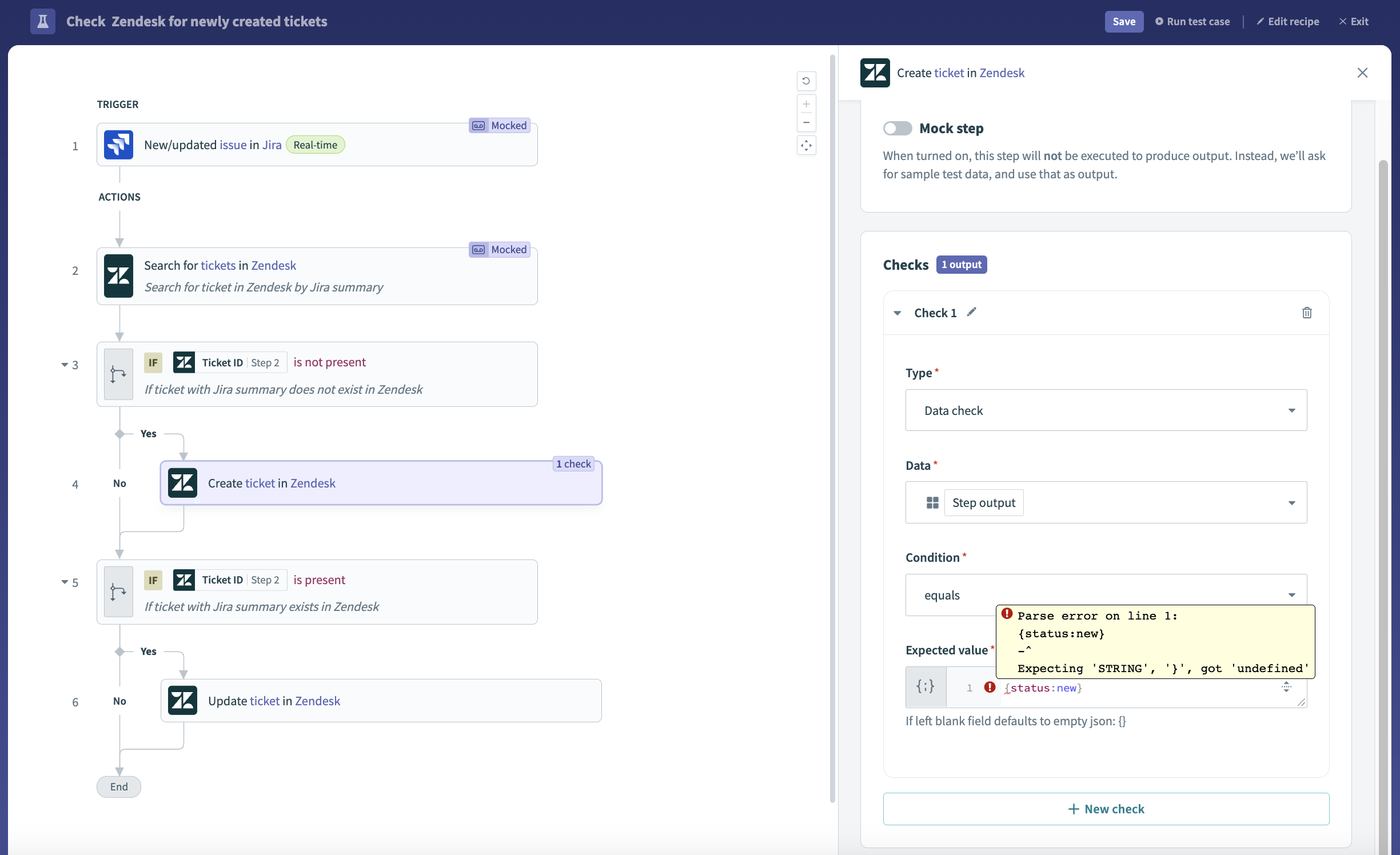This image is a screenshot from the Zendesk website showcasing a ticket management interface. At the top, there is a dark blue banner with text and buttons. On the far left, the banner displays the prompt, "Check Zendesk for newly created tickets." On the far right, buttons labeled "Save," "Run Test Case," "Edit Recipe," and "Exit" are visible.

Beneath the banner, within a white area, the word "Trigger" is prominently displayed. Below this, a sequence of steps is outlined:

1. "New updated issue in JIRA real-time."

Following the trigger, "Actions" are listed as follows:

2. "Search for tickets in Zendesk. Search for tickets in Zendesk by JIRA summary."

This step bifurcates based on ticket ID presence:

- If the ticket ID from step 2 is not present and the ticket with JIRA summary does not exist in Zendesk (Yes), the system will create a ticket in Zendesk.
- If the ticket ID from step 2 is present and the ticket with JIRA summary exists in Zendesk (Yes), the system will update the existing ticket in Zendesk. In both scenarios, a "No" condition leads to an endpoint labeled "End."

On the far right, a section titled "Create ticket in Zendesk" is visible along with a note stating "Mock step. When turned on this step will not be executed to produce output. Instead, we'll ask for sample test data and use that as output." Below this, a segment titled "Checks" lists "One output, Check one" with attributes such as "Type: Data check" and "Data: Step output. Condition equals Expected value."

A yellow text box partially obscures part of the text with the error message "Parse error on line one. Status new. Expecting string. Got undefined." Beneath this, there is a note stating, "If left blank, the field defaults to empty JSON."

At the bottom of the image is a white rectangle containing the option labeled "+ New Check."